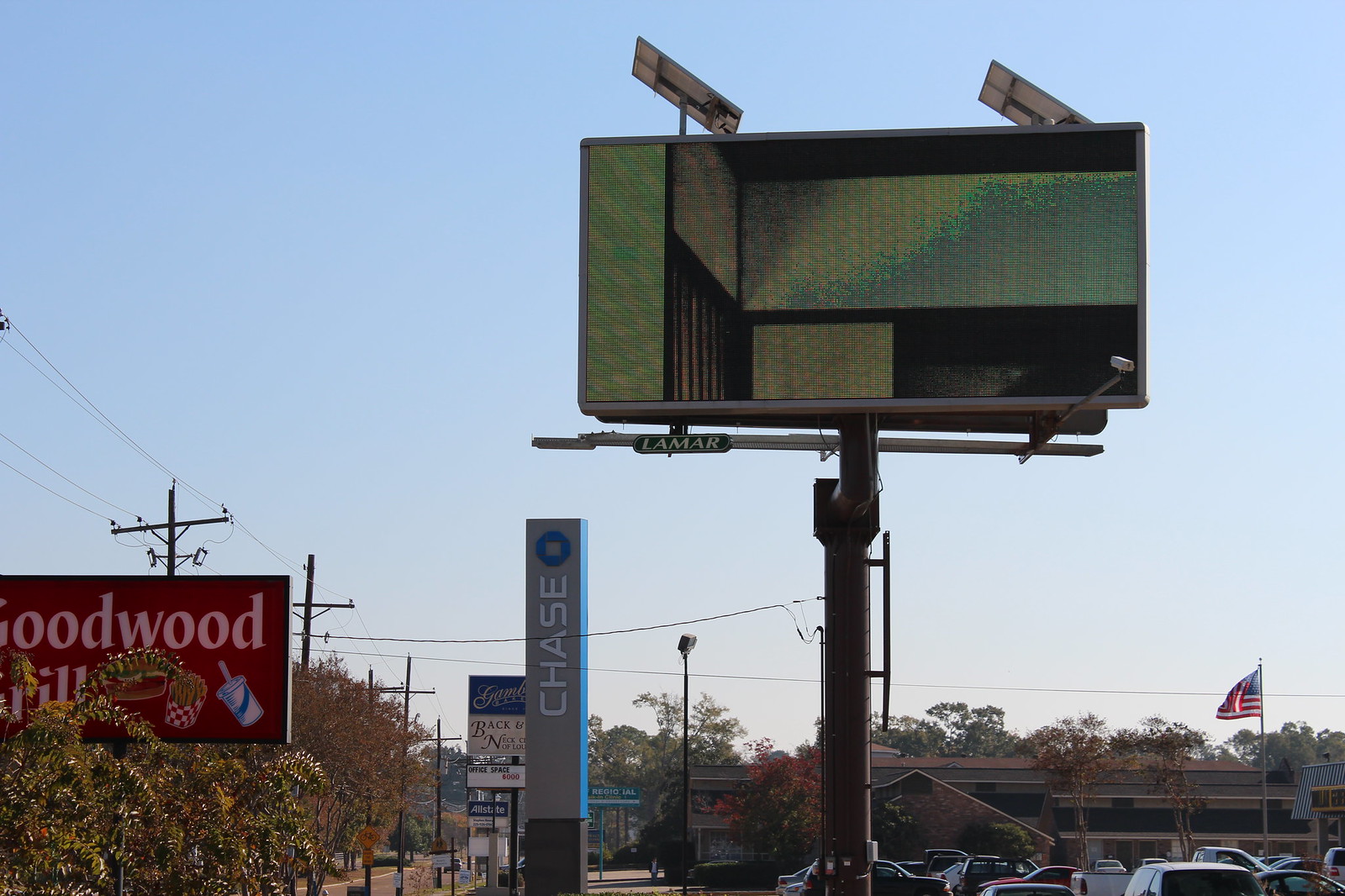The photograph showcases a large, blank billboard prominently situated in an outdoor retail park in America. The billboard, a dark jade green with some black and grey hues, dominates the top half of the image, mounted on a tall metal pole with visible support structures and the word "LAMAR" inscribed on the lower metal beam. Attached to this structure is a CCTV camera. Below the billboard, the scene unfolds into a mixed-use area featuring various signs and buildings. To the left, a partially obscured "Goodwood Grill" sign, with illustrations of a milkshake, fries, and a burger, hints at a restaurant presence. Nearby, a Chase Bank sign is visible, indicating the proximity of financial services. At the bottom right, an American flag waves above a parking lot filled with cars, bordered by trees and additional utility poles with overhead electrical cables stretching into the distance. The streets are lined with both commercial and possibly residential buildings, suggesting a typical American strip mall setting just off a main highway.